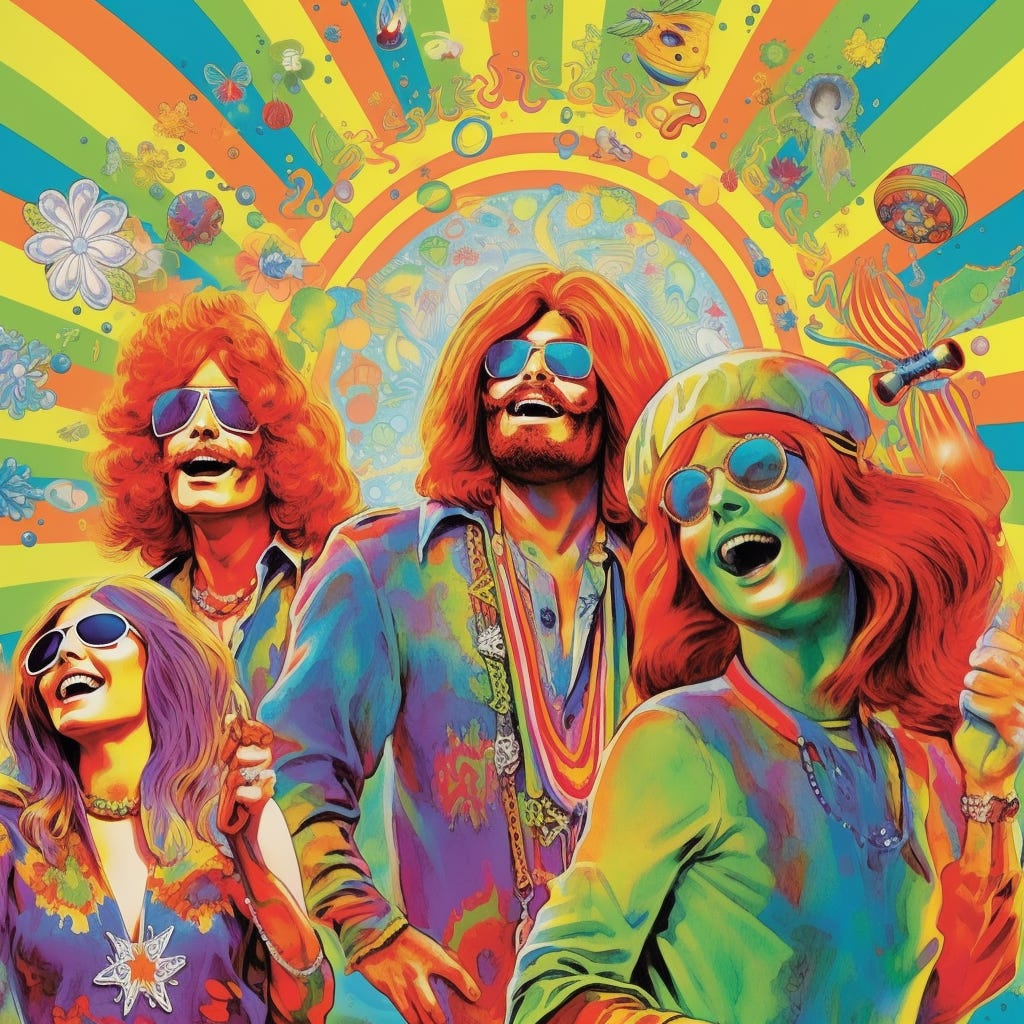The image is a vivid, psychedelic artwork or watercolor painting featuring four individuals dressed in quintessential 1970s-inspired outfits. Two men with red hair and two women, one with red hair under a French-looking hat and one with purple and blonde hair, are adorned in a mix of colorful tops—purple, blue, green, and flower-patterned. They all accessorize with long jewelry and beads, and wear sunglasses while standing vertically and looking upwards, seemingly singing or laughing with evident joy. The background is dominated by an artistically rendered sun, with rays displayed in a spectrum of green, orange, blue, and rainbow colors, adding to the vivid ambiance. The scene also includes floating objects like microphones, bubbles, and a butterfly in the upper right-hand corner, enhancing the '70s hippy vibe. The artwork creates an atmosphere reminiscent of a colorful store selling items like incense, capturing a sense of vibrant, carefree celebration.